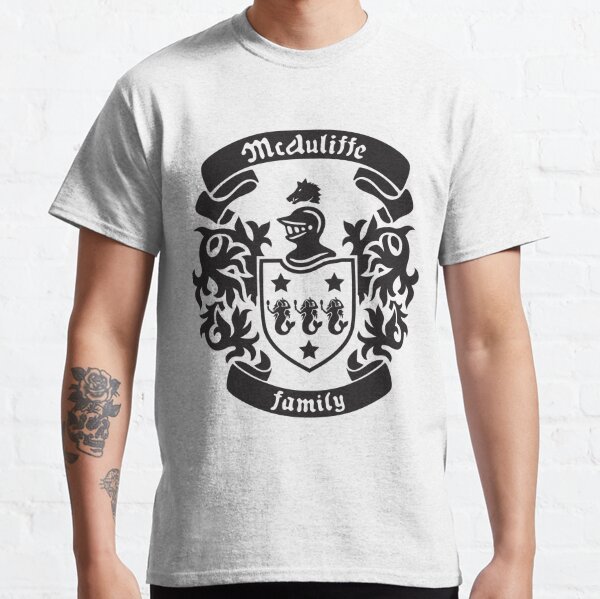This photograph features the torso of a Caucasian male model, prominently displaying a short-sleeved, light gray t-shirt. The focus is on the detailed design of the t-shirt rather than the individual, as the head is not visible. The t-shirt showcases a coat of arms for the McAuliffe family, with "McAuliffe" written at the top and "family" at the bottom in black banners. A distinct shield in the center is outlined in black with a white background and contains three black stars arranged in a triangular shape—two at the top and one at the bottom. Nestled between these stars are three black mermaids in a waving position. Above the shield, there's a knight's helmet illustrated in black. The model's right arm features a prominent tattoo of a skull entwined with roses, rendered in black ink. This t-shirt, possibly created for family reunions, combines traditional symbols and personalized elements, making it a distinctive piece of clothing.